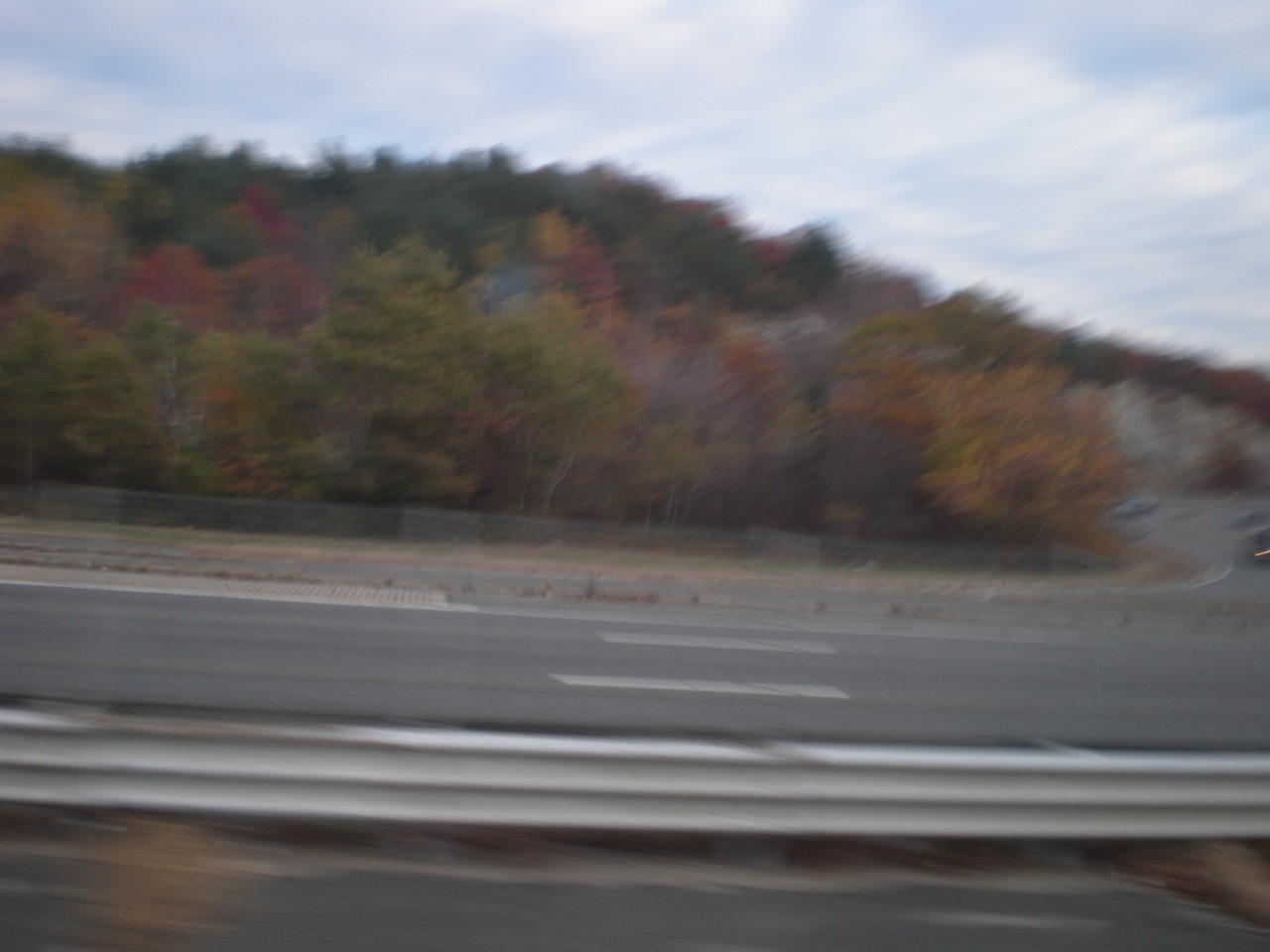This detailed, outdoor daytime photograph captures a slightly tilted, horizontal scene of a multi-lane highway bordered by various trees. The expansive light blue sky, interspersed with bright white clouds, occupies the top 15% of the image. Below the sky, there's a mixture of large trees exhibiting fall colors: predominantly dark green, interspersed with vibrant oranges, yellows, and reds, suggesting the photograph was taken in autumn. These trees, approximately one and a half to two stories tall, stand against a gentle, descending hill.

In the foreground, extending horizontally from the lower left to the lower right edge, there is a gray, three-lane highway marked with white horizontal lines. This highway is divided by a low metal bumper median. On the far side of the highway is a one-lane frontage road going each way, separated from the highway by a small chain-link fence. This frontage road contains a couple of dark, blurry cars towards the right. The photograph, likely taken from a moving vehicle out the left window, has a noticeable blur, particularly evident in the foreground and the metal crash barrier running along the highway. There are no words, text, or print visible in the image.